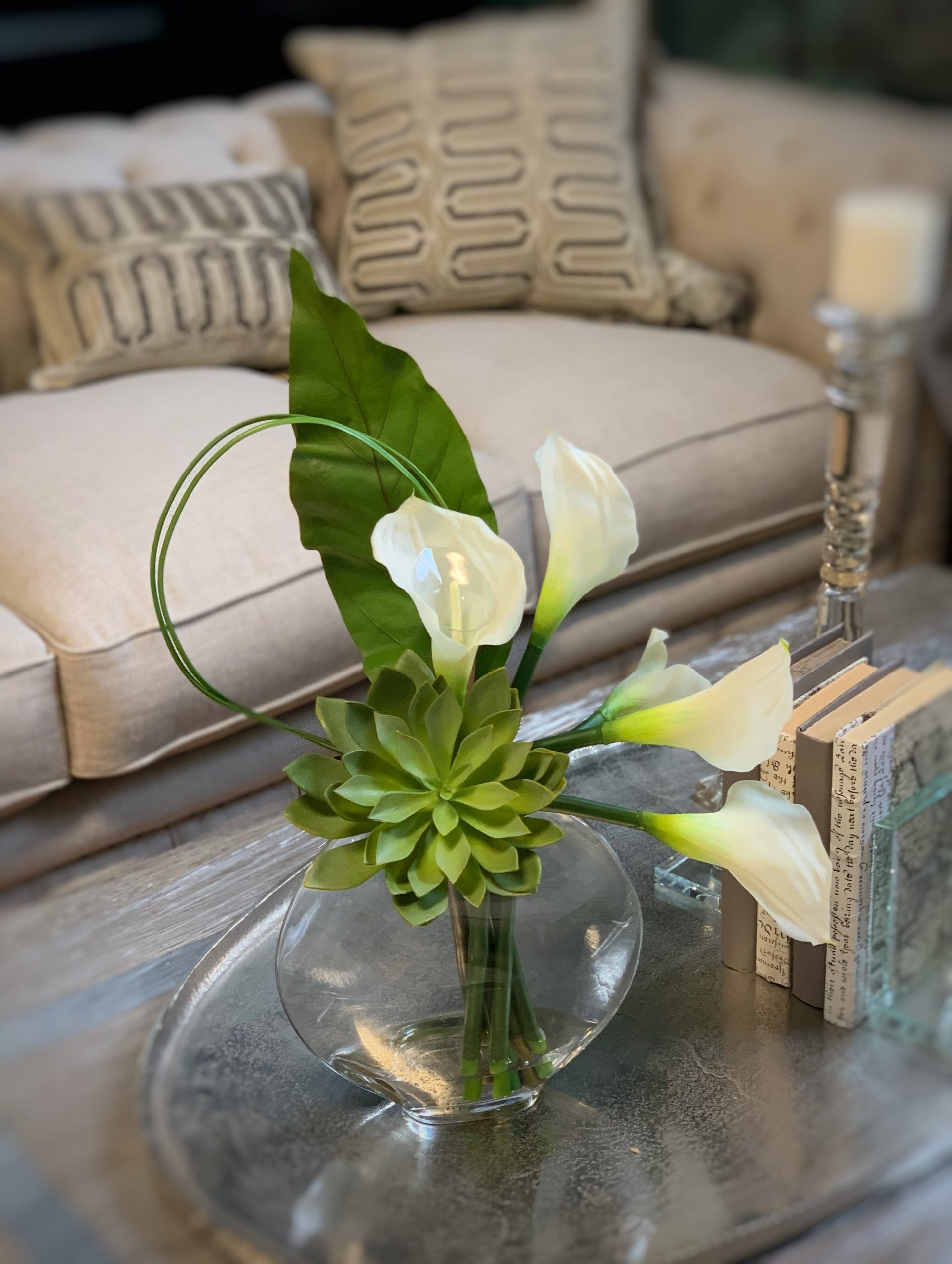This vertical rectangular photograph captures a formal, elegant living room. Dominating the background is a beige couch adorned with two decorative pillows featuring swirling, circular designs in dark brown. One pillow is vertical with two rows of the pattern, while the other, slightly larger with a square shape, features three rows of this design and rests turned on its side.

In front of the couch stands a distressed wood coffee table topped with an array of glass objects. Central among these is a clear, round glass vase holding white lily-like flowers, their green leaves and stems visible through the water. Additionally, a succulent-like plant with interconnecting leaves complements the flowers. To the right of the vase is a collection of three or four books, their bindings in shades of dark and light brown, held neatly in place by clear glass bookends. A tall, clear candle holder with a white candle stands out on the table, adding a touch of sophistication to the scene. The overall ambiance is one of tasteful refinement, showcasing a meticulously arranged living space.